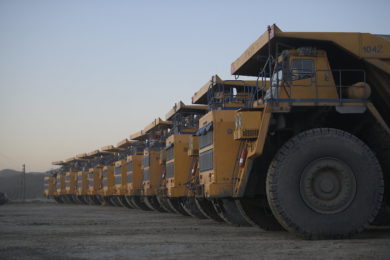This detailed color photograph, rectangular in shape, captures approximately a dozen large yellow dump trucks, likely water trucks, aligned in a perfectly neat horizontal row on a flat, dirt surface devoid of vegetation. These imposing vehicles, each with massive, dark tires and a uniform exterior, are reminiscent of equipment seen at mining sites. The front wheels and cabs of the trucks are distinctly visible, and you can see parts of their large dump beds towering over them. The scene is set against a backdrop that features a faint mountain range and a vast, open sky with a gradient blending from blue at the top to a subtle orange near the horizon, suggesting it might be either sunrise or sunset. The photograph, taken during a hazy and dim part of the day, portrays an expansive and rugged environment, emphasizing the grandeur and scale of the industrial machinery line-up.